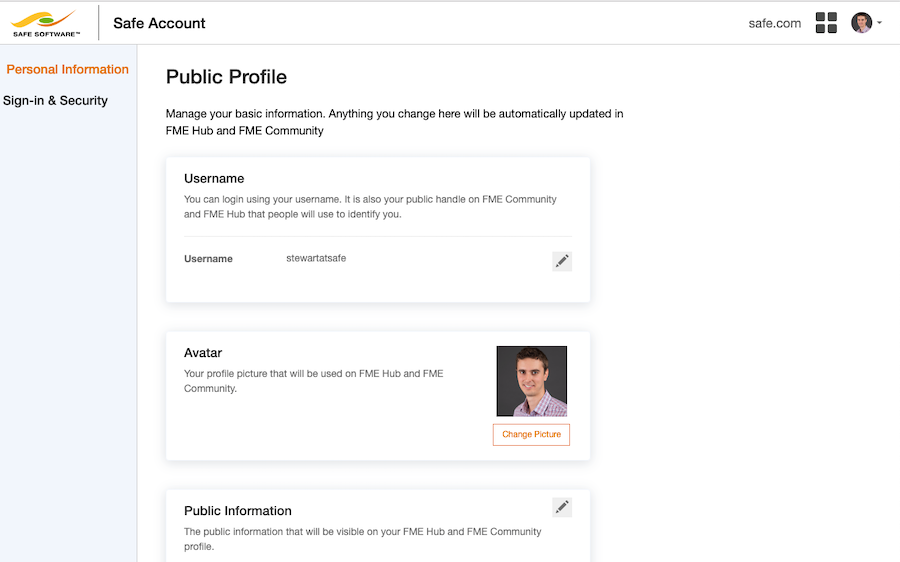### Descriptive Caption:

The image showcases the Safe Software website interface. In the upper left-hand corner, the Safe Software logo is prominently displayed alongside the text "Safe Software, TM." On the same row, the text "Safe Account" appears. To the far right of this row, there is the URL "safe.com" followed by a Microsoft symbol composed of four squares. Next to it is the profile icon of the user, accompanied by a drop-down menu indicated by an upside-down triangle.

Further to the left side of the page, several tabs are listed: "Personal Information," "Categories," and "Sign-In and Security," along with a "Public Profile" section. The Public Profile section provides a message informing users that any changes they make will automatically be updated in the FME Hub and the FME Community.

Beneath the Public Profile section, there are three separate rectangular boxes. The first box is labeled "Username," which states that users can log in using this username, also serving as their public handle on the FME Hub and FME Community. The sample username "stewardatsafe" is provided, accompanied by a pencil icon for editing. 

The second box features the user's avatar—a profile picture that will be utilized on both the FME Hub and the FME Community. The avatar is an image of a white man with brown hair, wearing a long-sleeve checkered shirt. A "Change Picture" button is located just below this avatar.

The final rectangular box displays "Public Information," which contains the details that will be publicly visible on the user's FME Hub and FME Community profile.